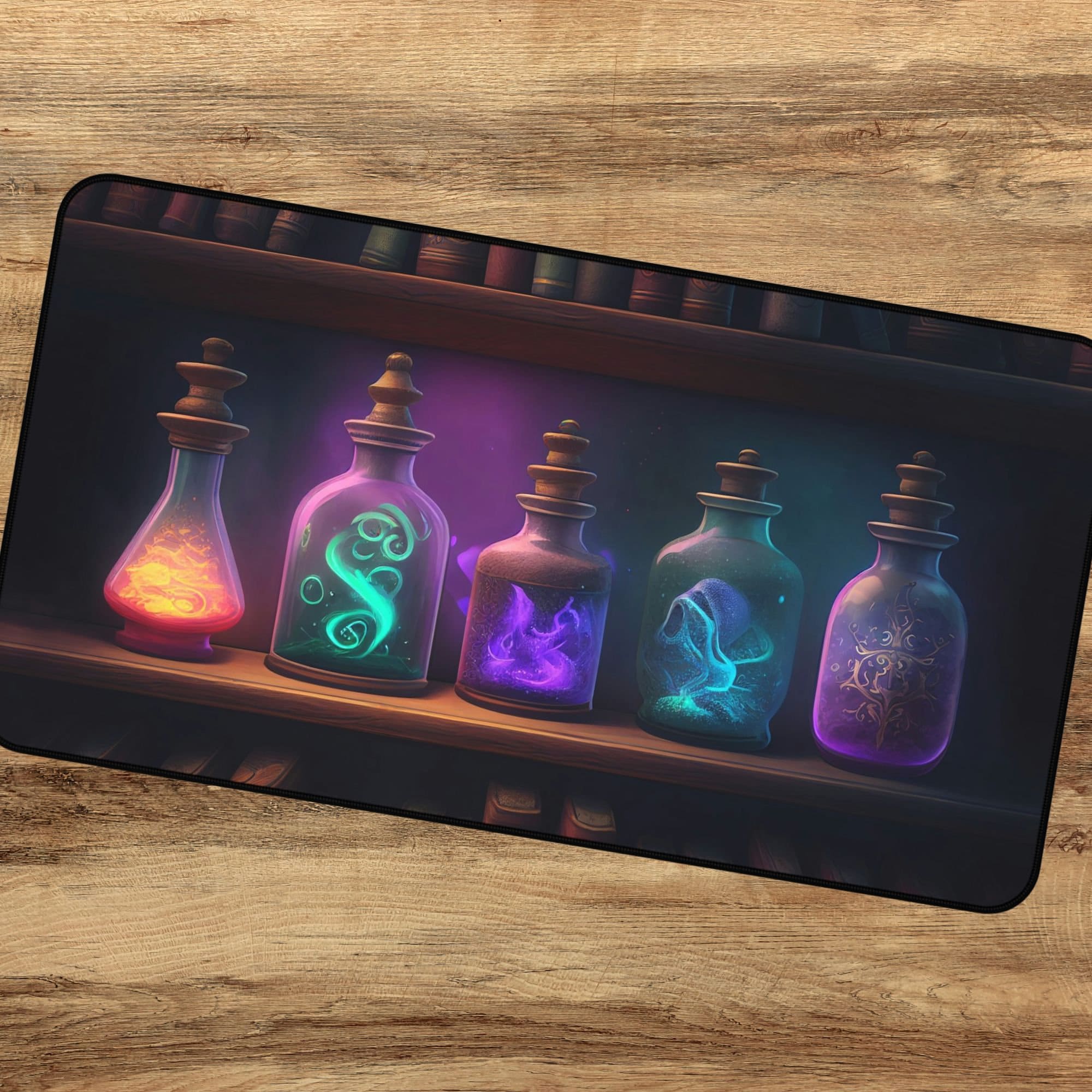In the image, a sleek black rectangular tablet rests on a wooden table. The tablet displays a detailed, computer-generated image of five distinct glass bottles placed on a shelf. The screen reveals an animated scene that features these bottles, each plugged at the top and exhibiting different shapes akin to scientific beakers or flasks. The bottles contain various colored elements: fiery orange-red substance, blue swirls, and purple mist or steam. Specifically, two bottles are filled with purple contents, two with light blue, and one with an orange-red fiery element. The image evokes a mystical or magical theme reminiscent of potions. Above the bottles on the shelf are book spines, while the tops of additional books are visible below them. Each bottle is unique, with one green potion emitting swirls and another glowing with purple light, adding to the enchanted atmosphere of the scene.